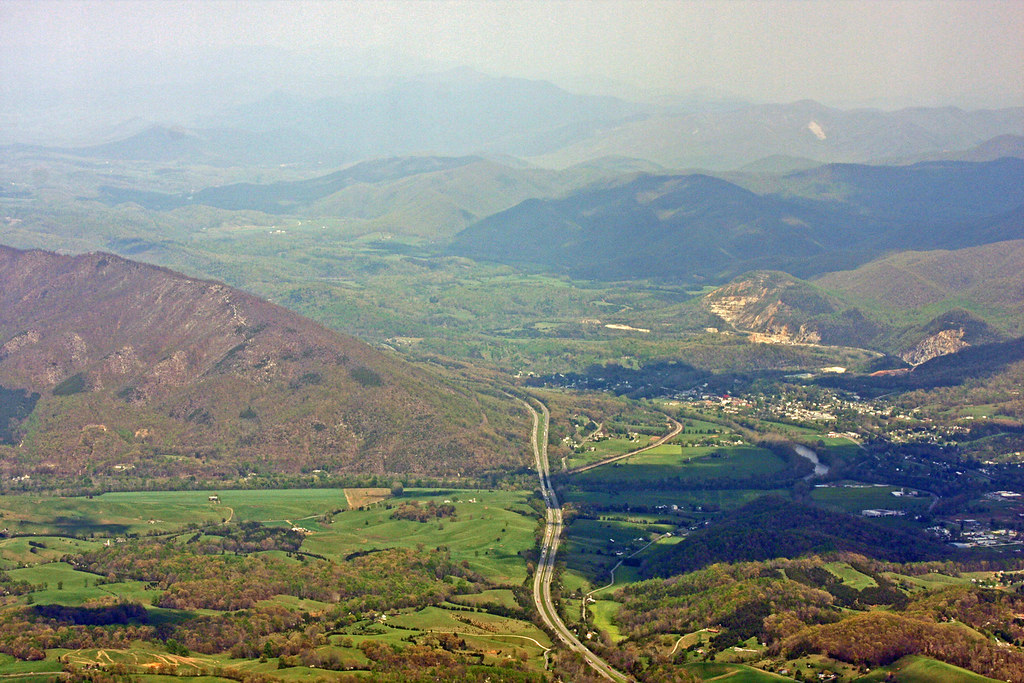This image, likely taken from a high vantage point such as a mountain or airplane, provides a breathtaking aerial view of a lush, vibrant landscape dominated by rolling hills and expansive fields. Central to the scene is a prominent four-lane highway with visible traffic flowing in both directions, accompanied by smaller roads branching off towards sparse, barely discernible housing areas. To the left, a substantial, rugged mountain rises with brown and rocky outcrops, flanked by several other hills and mountains that stretch across the backdrop. These distant peaks are partially shrouded in an overcast cloud cover, creating a misty, slightly obscured horizon. The right side of the image features a shaded area over smaller hills, cast by larger unseen formations beyond the frame. In the lower part of the image, the landscape transitions into a patchwork of vibrant green grass, fields, trees, and possibly farmland, with a small creek winding its way through on the right. There might even be tiny, indistinct dots that could be livestock grazing in the field. Overall, the photograph captures a serene and picturesque valley landscape with a harmonious blend of natural features and minimal human development.